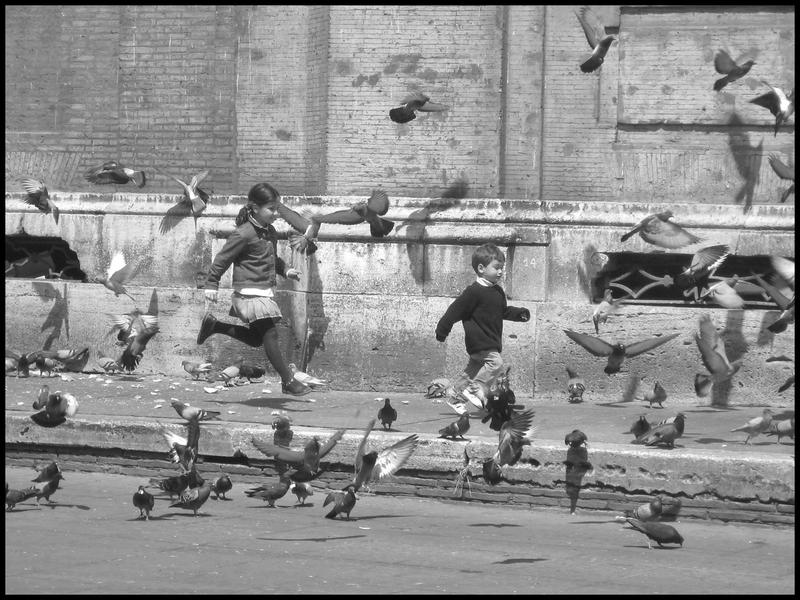In this evocative black and white photograph, a young boy in a sweater and a slightly older girl with a ponytail, wearing a skirt and a button-down jacket, are captured running down a city sidewalk surrounded by a flurry of pigeons. The children, with joyful enthusiasm, charge forward amidst the birds, some of which are perched on the pavement while others take flight. The scene is set against the backdrop of a tall brick building with a large stone foundation, adding a historical charm to the image. The steep curb leads to a layered brick masonry that drops off to the street, emphasizing the urban environment. Feathers are scattered across the sidewalk, heightening the dynamic motion of the image. The photograph, likely an old one, perfectly captures a moment of carefree childhood amidst the bustling life of the city.